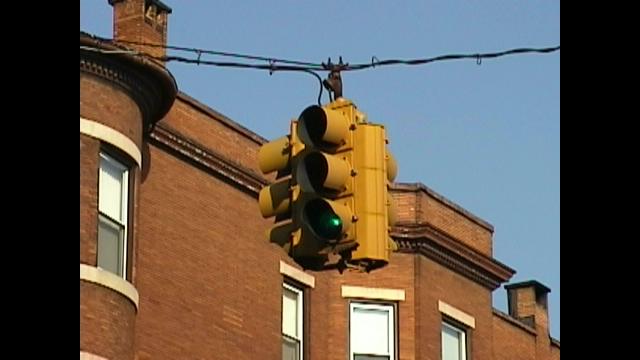This rectangular color photograph, bordered on both sides by fairly wide black panels, captures a scene viewed from the ground looking upward during the daytime. Dominating the center of the image is a yellow, triple-sided, three-way streetlight with the bottom light illuminated green, suggesting it is situated at a crossroad. The streetlight hangs from long, black, twisted wires extending horizontally across the frame. In the background on the left side, a large brick building with Victorian architectural features is visible. This dark red building likely serves as a residential apartment complex and showcases a combination of curved, tower-like shapes, long rectangular windows with yellow borders, and two chimneys extending from its roof. The solid light grayish-blue sky forms the backdrop, enhancing the clarity of the building’s and streetlight's details in this upward-looking view.